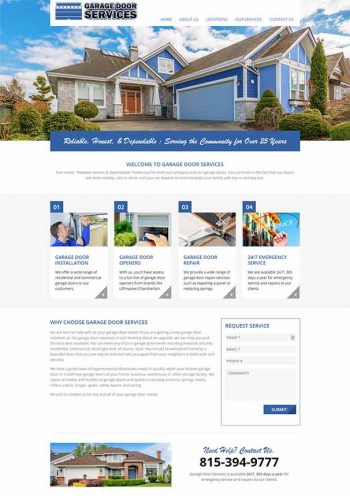The image features a promotional material for a company specializing in garage door services. Dominating the scene is a striking blue house that blends seamlessly with the equally vivid blue sky, punctuated by fluffy white clouds. The property is beautifully landscaped with evergreen shrubs adding a touch of greenery.

At the top of the image, within a blue box, there is some text indicating the company's longevity, stating "Serving the community for over 25 years," written in elegant script.

The banner welcomes you to "Garage Door Services" and provides further details in small print, which are not clearly legible. Below this section, four neatly organized blue boxes are numbered, highlighting the various services offered: 
1. Garage Door Installation
2. Garage Door Openers
3. Garage Door Repair
4. 24/7 Emergency Service

Farther down, a white section with the headline "Why Choose Garage Door Services?" is displayed in blue text, accompanied by two paragraphs of descriptive information written in black text. Adjacent to this, there is a gray-outlined form titled "Request Service," featuring input fields for customer details and a blue "Submit" button at the bottom.

Finally, the bottom of the page showcases another house with a friendly prompt, "Need Help?" followed by a contact phone number for immediate assistance.